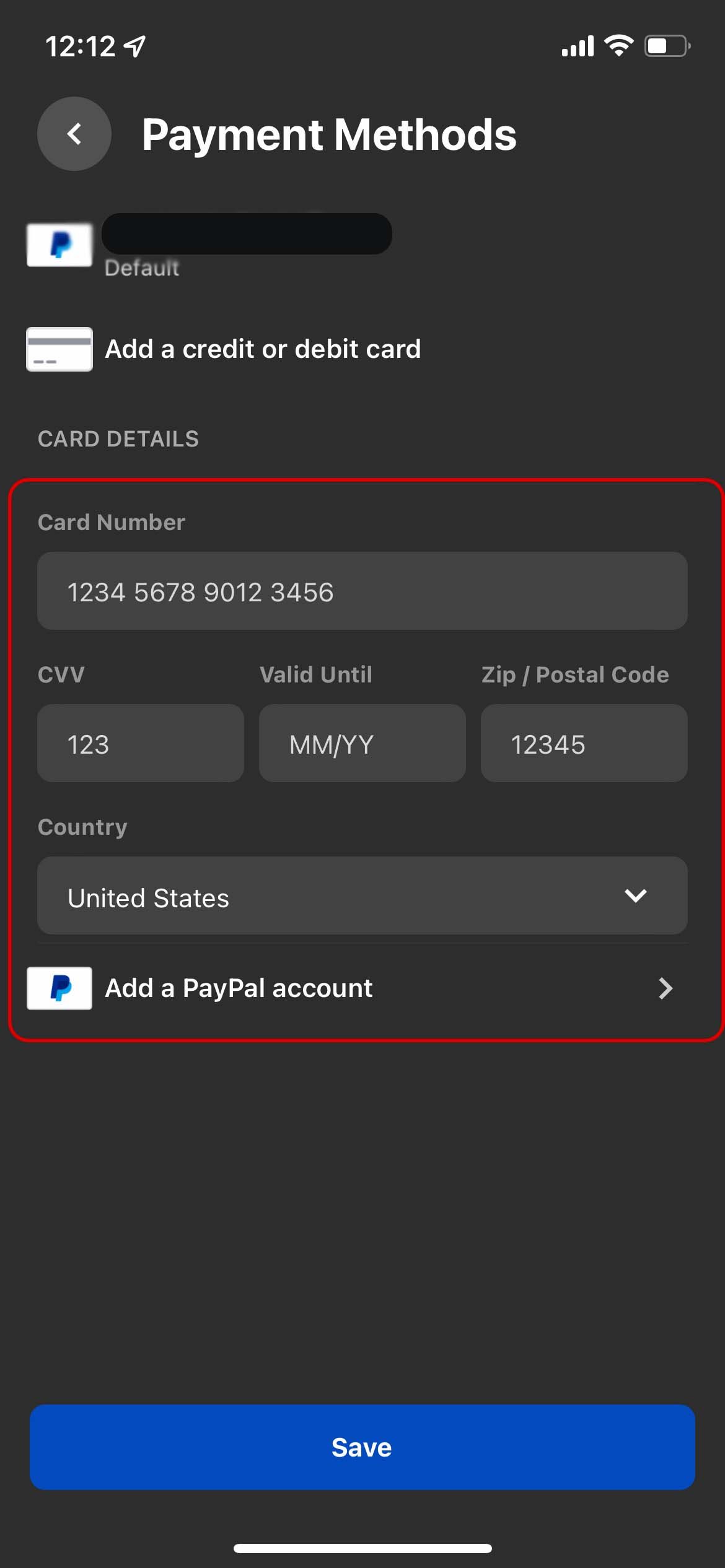The image is a vertically oriented mobile screenshot depicting a payment page with a uniform dark gray background. At the top, the status bar is visible: the time reads 12:12 on the left, while on the right, there are four cellular bars, a Wi-Fi icon, and a half-charged battery indicator. Below, the title "Payment Methods" is displayed prominently.

The first section lists the default payment method, marked with a PayPal logo on the left. The card number associated with this PayPal account is obscured by a black marker effect for security reasons. Beneath this, an option to "Add a credit or debit card" is presented in white text, accompanied by a white credit card icon featuring a horizontal gray stripe.

Further down, there is a section titled "Card Details," framed by a red-bordered rectangle. Inside this section, placeholder card information is listed: card number "1234 5678 9012 3456," CVV "123," expiration date "MM/YY," zip/postal code "12345," and the country "United States." At the bottom of the page, there's an option to add a PayPal account again, indicated by another PayPal logo. The interface concludes with a prominent blue "Save" button.

This detailed layout helps users manage and add new payment methods with visual clarity and ease.